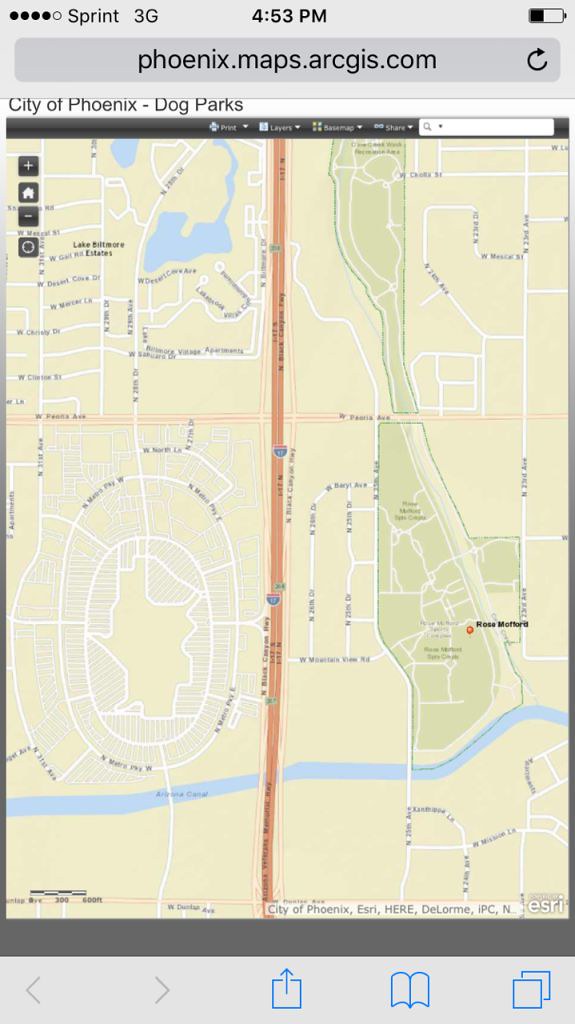The image is a phone screenshot prominently displaying a map of Phoenix dog parks. At the top center of the screen, the time is shown as 4:53 PM. To the right, the battery icon indicates that the battery is slightly below halfway charged. On the left, the network information shows "Sprint 3G" with four out of five signal bars. The URL in focus is "phoenix.maps.arcus.com."

Central to the image is a detailed map labeled "City of Phoenix Dog Parks." The map is filled with text, much of it too small to be legible. Running vertically through the center of the map is an orange highway. Near the top, just above the center, a lighter orange road is visible, running horizontally. Towards the bottom, a blue line, representing a river, spans horizontally across the entire width of the map. On the left side of the image, there are circular patterns likely indicating a complex road network or roundabouts. Conversely, areas on the right side are highlighted in green, possibly denoting park areas or green spaces. At the bottom right of the image, text reads "City of Phoenix, Esri, Delorme IPCN."